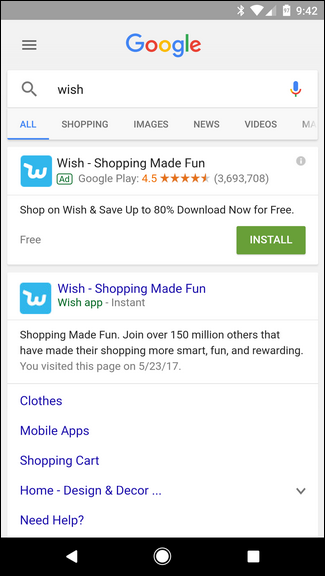This image is a screenshot of a Google search result page. At the top, the Google logo is prominently displayed followed by the search query "wish." The search results highlight the Wish shopping platform with the tagline "Wish Shopping Made Fun." The page encourages users to shop on Wish by stating, "Shop on Wish and save up to 80%. Download now for free. Install." It also reiterates, "Wish: Shopping Made Fun," emphasizing the user-friendly and enjoyable experience. The description further notes that over 150 million people have joined Wish, making their shopping experience smarter, more fun, and rewarding. At the bottom, the screenshot illustrates a variety of categories available on Wish such as clothes, mobile apps, shopping carts, home design, and decor. Additionally, there is a prompt offering help at the end of the search results.